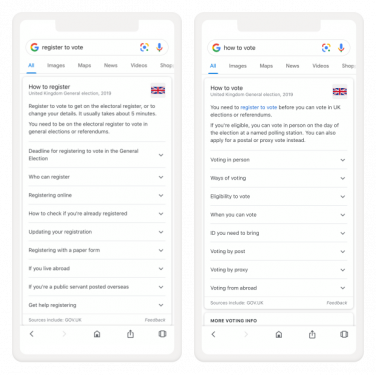The image shows two smartphone screenshots placed side by side, each displaying a Google search results page against a white background. 

On the left-hand side, the search query in the top box reads "register to vote." The familiar Google logo, marked by the letter "G," is prominently displayed next to a blue microphone icon and the Google Lens icon, characterized by a small square in Google colors. Below the search bar, the first result is titled "How to register," followed by several lines of text, although the small font renders the specific details unreadable. Additional search results appear below, each accompanied by a dropdown arrow indicating expandable content.

On the right-hand side, the search query reads "how to vote." Similar to the previous screenshot, the leading search result is titled "How to vote," accompanied by several lines of text, which are also too small to decipher. Further search results follow, each featuring a similar dropdown arrow for additional information.

Both screenshots provide a quick glimpse into Google's search interface and display important information on voting procedures, though the specific contents are not legible due to the small font size.